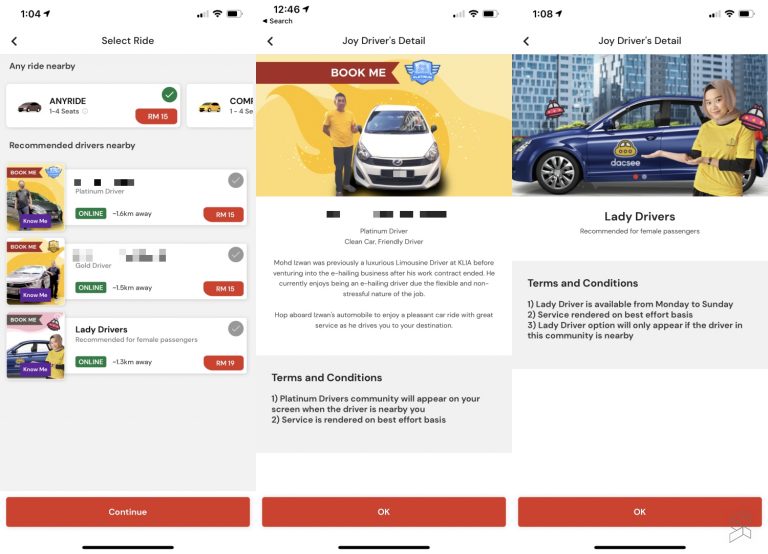The image features three side-by-side screenshots taken on a mobile phone, each displaying details from a ride-hailing app at different times of the day.

**Screenshot 1 (Time: 1:00 PM)**
- **Heading:** "Select a Ride"
- **Subtitle:** "Any Ride Nearby, Any Ride, 1-4 Seats"
- **Status Indicator:** Green tick
- **Additional Details:** "R.A.M. 15 before" (ambiguous information)
- **Icons:** Little yellow car with partial text starting with "C.O.M." (likely indicating “Compact”)
- **Driver Options:**
  - **Option 1:** 
    - **Picture:** Blurry image of a person standing in front of a car
    - **Status:** "Book Me"
    - **Driver Rating:** Platinum Driver 
    - **Distance:** 1.6 kilometers away 
    - **Remark:** "R.A.M. 15"
    - **Note:** Grayed-out ticks to the right
  - **Option 2:**
    - **Picture:** Person standing next to a silver car, car on the left, person on the right
    - **Status:** "Book Me"
    - **Driver Rating:** Gold Driver
    - **Distance:** 1.5 kilometers away
    - **Remark:** "R.A.M. 15"
  - **Option 3:**
    - **Picture:** Female standing in front of a blue car
    - **Status:** "Book Me" (grayed-out)
    - **Special Note:** "Lady Drivers Recommended for Female Passengers"
    - **Distance:** 1.3 kilometers away

**Screenshot 2 (Time: 12:46 PM)**
- **Heading:** "Joy Drivers Detail"
- **Driver Information:**
  - **Picture:** Male in a yellow shirt and gray pants standing next to a white car (person on the left, car on the right)
  - **Status:** "Book Me"
  - **Rating:** Platinum Driver
  - **Special Features:** Clean Car, Friendly Driver
  - **Driver Name:** "Mohd" 
  - **Additional Background:** Former luxurious limousine driver at an airport (KLIA/KLJA, unclear due to blurriness), now an e-hailing driver enjoying the flexibility and low stress
  - **Narrative:** Encourages users to enjoy a pleasant ride with great service
- **Terms and Conditions:** 
  1. Platinum Drivers Community will appear on your screen when the driver is nearby.
  2. Service is rendered on a best effort basis.
- **Action Button:** Red "OK" button

**Screenshot 3 (Time: 1:08 PM)**
- **Heading:** "Joy Drivers Detail"
- **Driver Information:**
  - **Picture:** Female standing in front of a blue car (car facing left, female at the rear right, gesturing towards the car)
  - **Clothing:** Yellow short-sleeved shirt with black long sleeves underneath and a beige hijab
  - **Status:** "Lady Drivers, recommended for female passengers."
- **Terms and Conditions:** 
  1. Lady Driver is available from Monday to Sunday.
  2. Service rendered on a best effort basis.
  3. Lady Driver option will only appear if a driver from this community is nearby.
- **Action Button:** Red "OK" button

No other text or images are present in the screenshots.